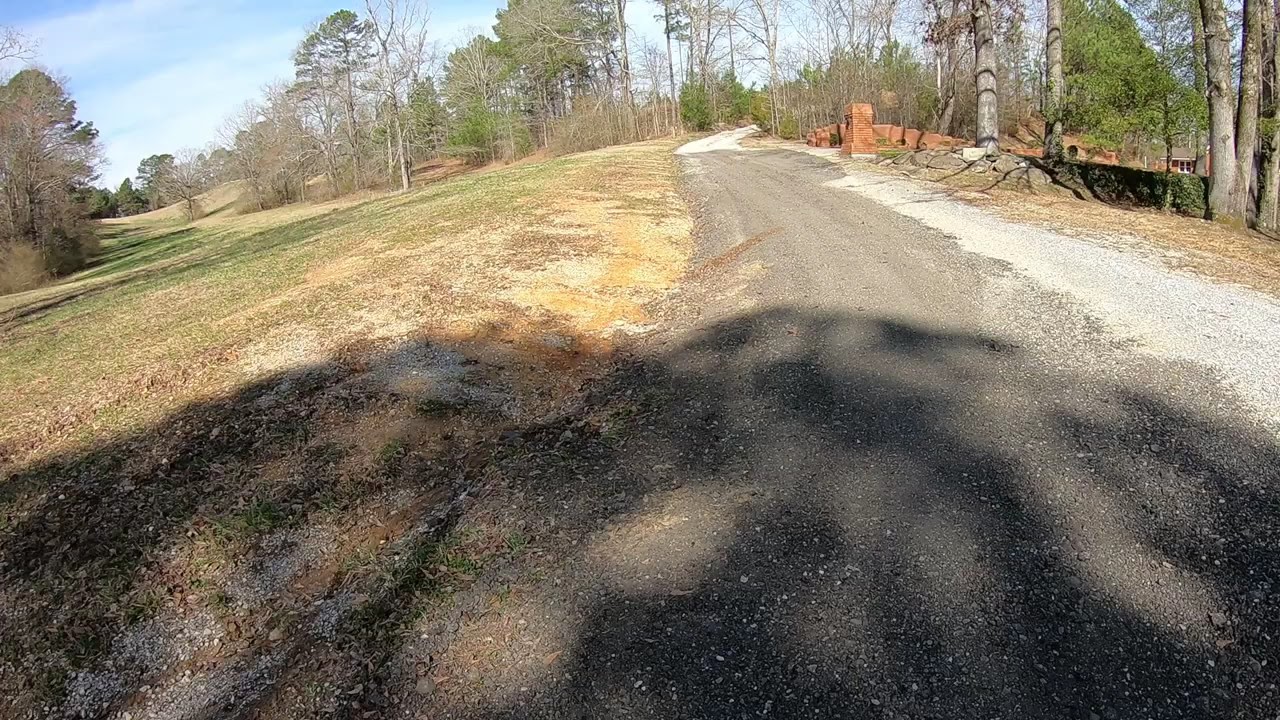This outdoor photo captures a narrow gravel lane, seemingly transitioning into a mixed asphalt surface, under a partly cloudy, blue sky. The road stretches from the lower left foreground to the center-right, flanked by a distinct shadow likely cast by a tree with sparse, late fall or early winter foliage. To the left of the lane, a patchy field of dying grass with brown and yellow hues slopes downward slightly, transitioning into a tree line of mostly bare trees. The distant trees enclose the scene, adding to the sense of seasonal change. The right side of the lane features a distant brick wall, more gravel, and patches of dirt, with tall trees emerging in the background. The landscape reflects a serene and somewhat desolate countryside ambiance.